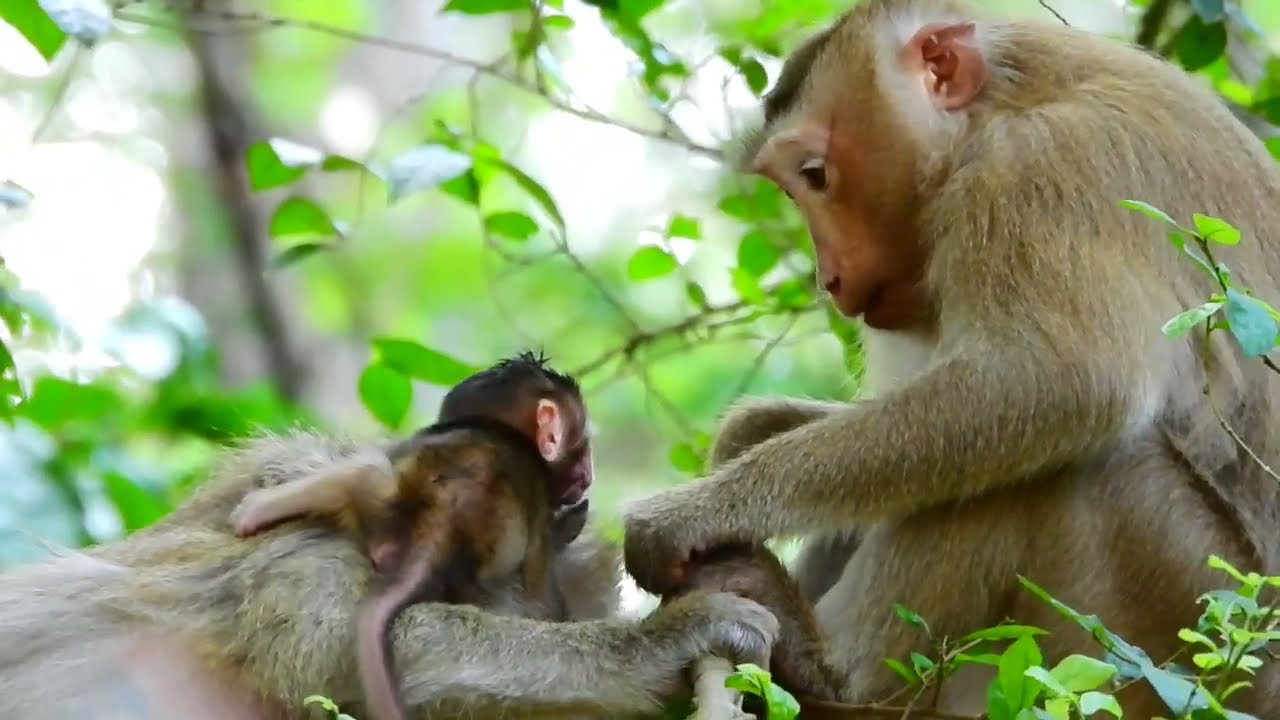This captivating outdoor photograph captures a serene moment high in the treetops where three monkeys are seen amidst the greenery. The prominent adult monkey on the right has light brown fur and distinctive pink, elvish ears, gazing downwards with a surprised expression. A playful, dark brown-furred baby monkey, with less fur and a long pink tail, is perched on the back of another adult monkey. The baby's large pink ears stand out as it faces away from us, giving a glimpse of its back. Encircling these adorable primates are vivid green leaves and branches, with sunlight filtering through, illustrating a bright daytime setting. The background is artfully blurred, ensuring the focus remains on the intimate interaction between the monkeys.